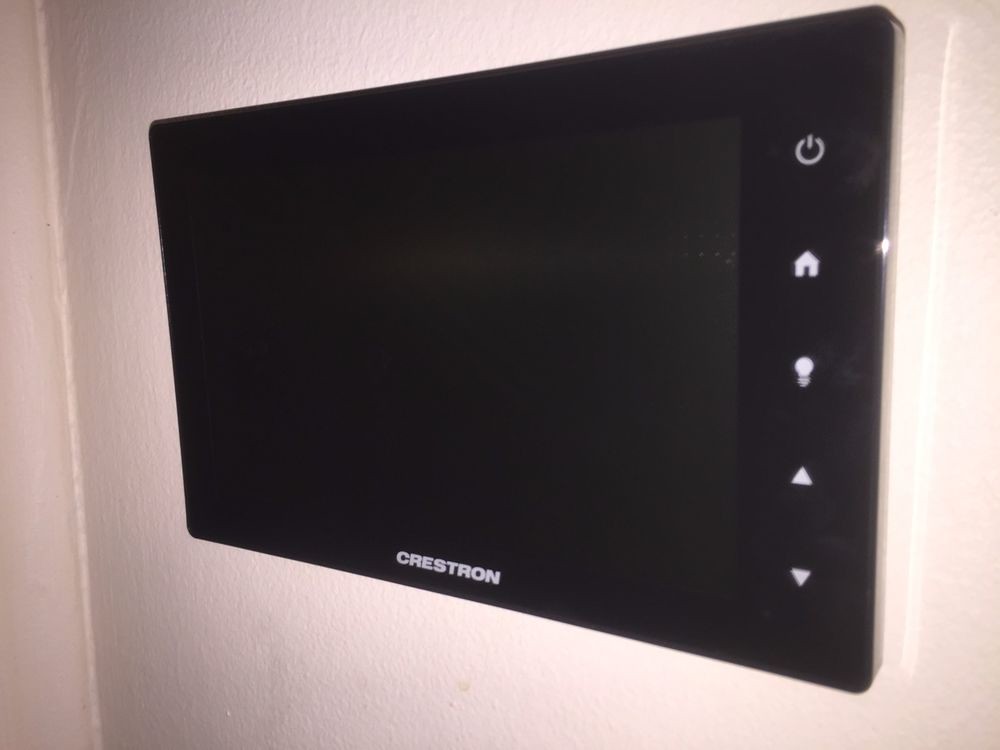This color photograph captures a minimalist scene dominated by a stark white wall. The image is shot at an angle, revealing the corner of the wall on the left side. The central focus is a sleek, black, rectangular screen encased in a matching black frame. The screen is currently off, displaying no content. Below the screen, the brand name "CRESTRON" is printed in crisp white lettering.

To the extreme right of the screen, a vertically aligned control panel is visible, featuring five distinct icons from top to bottom: a power button, a home symbol, a light bulb, and two directional arrows pointing up and down, respectively. Near this control panel, light hits a corner of the black screen, casting a subtle reflection on the adjacent wall, adding a touch of depth to the otherwise straightforward composition. The photograph is devoid of any human or animal presence, focusing solely on the device and its surroundings.